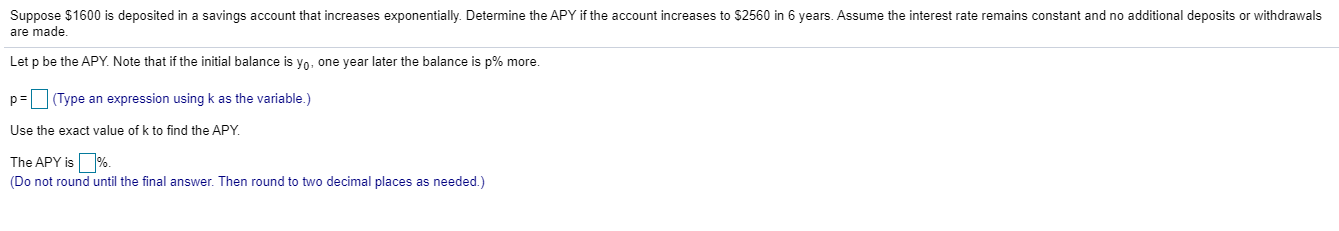This is a detailed screenshot of a website displaying a homework question related to economics or accounting on a stark white background. The homework problem is presented at the top of the page and reads as follows: "Suppose $1,600 is deposited in a savings account that increases exponentially. Determine the APY if the account increases to $2,560 in 6 years. Assume the interest rate remains constant and no additional deposits or withdrawals are made." Underneath this question is a thin gray line that separates it from further instructions below.

The next section begins with, "Let P be the APY," followed by a detailed explanation of the problem. It states, "Note that if the initial balance is Y sub G, one year later, the balance is P percent more." This is immediately followed by "P equals," and then an empty text box, prompting the student to enter their answer. Further instructions advise the student to "Type an expression using K as the variable, and then beneath this, use the exact value of K to find the APY."

Another empty text box labeled "The APY is ______ percent" follows. Below this line, there is a note in blue text that reads, "Do not round until the final answer. Then round to two decimal places as needed." Both text boxes, as well as the text line next to the "P equals" section, are highlighted in blue, indicating areas where the student is required to input their answers.

The bottom of the page features a significant amount of negative space, emphasizing the simplicity and focus on the economics or accounting problem presented at the top.

In summary, the screenshot depicts an exercise in determining the Annual Percentage Yield (APY) for a savings account given a specific problem scenario, with inputs required from the student in various highlighted fields.